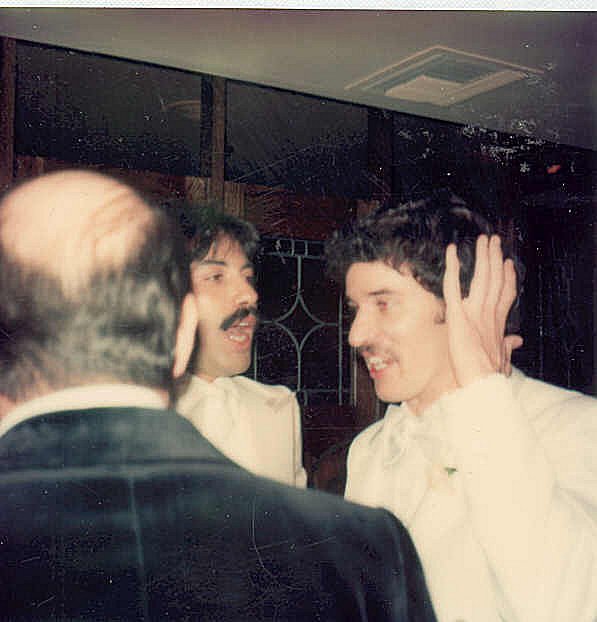This vintage photograph appears to have been scanned and shows a lively moment captured, likely from several decades ago. In the center, there is a man who strongly resembles actor and comedian Freddie Prinze Sr., father of Freddie Prinze Jr. He has short black hair, a black mustache, and appears to be speaking with his mouth open to a person to his right. Both of these central figures are dressed in white tuxedos with white bow ties. The man to the right is engaged in conversation, possibly covering his ear either out of habit or due to the noise.

To the left of Freddie Prinze Sr. stands a man with male pattern baldness, having brown hair around the sides. He is wearing a black suit jacket paired with a white collared shirt. The setting suggests an indoor environment, possibly a restaurant, highlighted by the presence of a ceiling vent and windows in the background, indicating a structured and somewhat formal venue. The photograph is slightly hazy, adding to its nostalgic feel. The man central to the conversation might be Tony Orlando, identifiable by his mustache and hair parted in the middle, who seems to be vocalizing loudly but not in anger. The skin tones of the individuals are fairly light, eliminating the possibility that they are African American. Overall, this snapshot captures a dynamic exchange among three men, amidst a nostalgically formal setting.